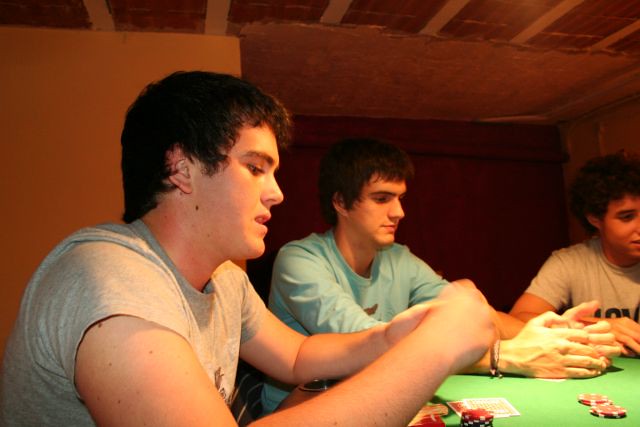The image features three young men, all with brown hair, seated around a green table, likely covered with a green tablecloth. They appear to be playing a card game, each holding their cards and covering them with their hands. There are poker chips, primarily red and white, scattered on the table, along with a dice. The young men are positioned with one on the left, one in the center, and the third partially visible on the right. Attire includes two wearing gray t-shirts and one in a long-sleeved light blue shirt. The background suggests a basement setting with brownish wood-paneled walls. The overall scene captures a casual indoor game of cards among teenagers.